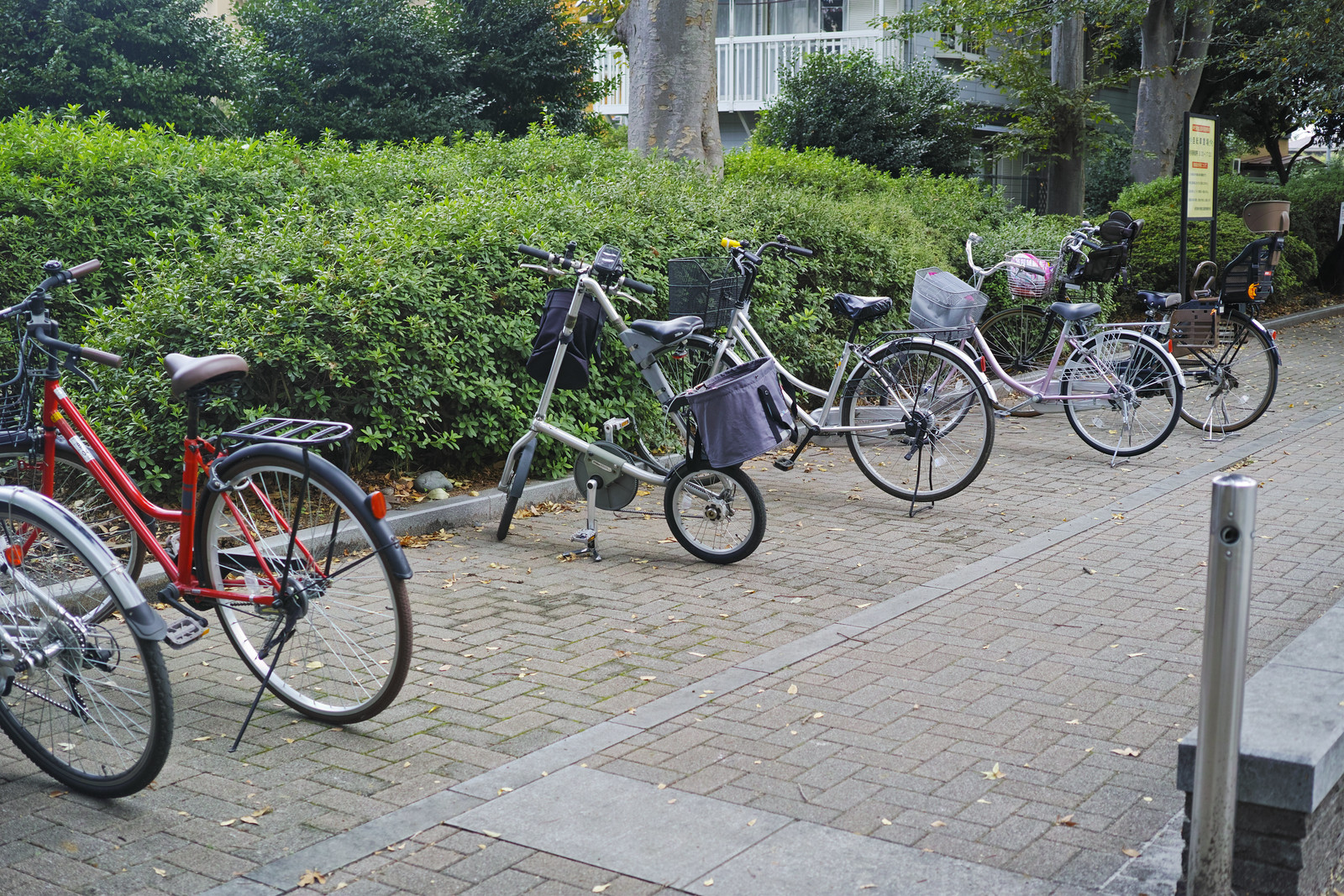In this outdoor photograph, a brick pathway hosts a lineup of six distinct bicycles, arranged perpendicular to the curb. The pathway itself, composed of patterned bricks, shows signs of green moss and weeds growing through the cracks. Among the bicycles, one is a red and black model, another is uniquely shaped with a triangle frame and a small basket at the back. There's also a gray bike with a black seat featuring a front basket, a white bike with a white basket, a pink girl's bike with pink handles, and a black men's bike with a baby seat. Two of the bicycles are noted to have children’s seats, while a couple have front baskets for carrying items. This scene is framed by lush green bushes and trees, with a glimpse of a two-story gray house featuring a white porch and railing in the background. The photo is reminiscent of a grayish day, adding a calm atmosphere to this snapshot of everyday life.